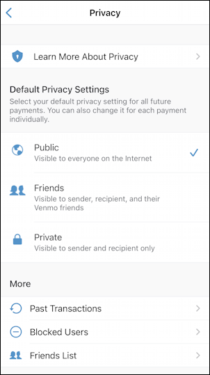This detailed screen capture showcases a privacy settings page, likely from a mobile app or web platform. The image is encapsulated by a black border. 

At the very top, a white bar features a blue back arrow and the title "Privacy" in black font. Below this heading, a horizontal gray line divides the screen, followed by an empty gray bar.

Further down, a white bar presents a blue shield icon accompanied by black text reading "Learn more about privacy." 

Continuing downward, the screen is sectioned into a gray area labeled "Default Privacy Settings." Here, explanatory text reads: "Select your default privacy settings for all future payments. You can also change it for each payment individually."

Beneath this section, three white options are separated by thin gray lines:
1. **Public**: Marked by a blue globe icon and a blue check mark, this setting is described as "Visible to everyone on the internet."
2. **Friends**: Illustrated with two cartoon people icons, this option notes, "Visible to sender, recipient, and their Venmo friends."
3. **Private**: Symbolized with a blue padlock icon, this setting states, "Visible to sender and recipient only."

Following these options, another gray section labeled "More" includes:
- **Past Transactions**: Denoted with black text and a blue circle.
- **Blocked Users**: Indicated by a blue circle with a slash and black text.
- **Friends List**: Characterized by two blue person icons and black text.

Each item in this section has a small gray arrow beside it to expand the menu.

The image quality is exceptionally clear, ensuring the text and icons are easily readable.